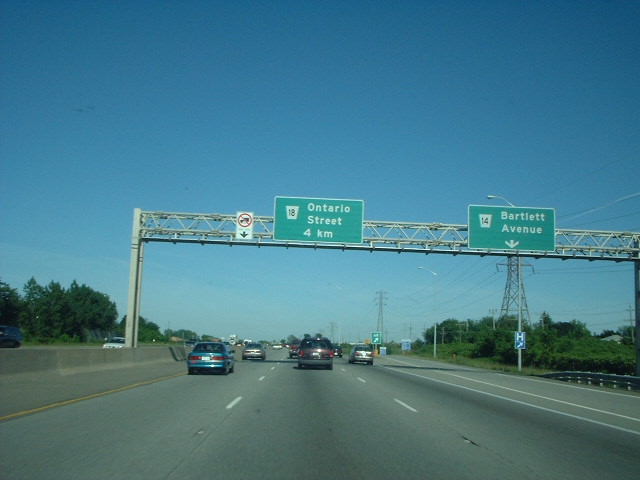The image captures a bright and sunny day on a busy three-lane highway, taken from the center lane of the roadway. Overhead, there are several highway signs attached to metal posts. The leftmost sign is a small white rectangle indicating "no trucks" for the left lane. To the right are two large green signs with white text: the left one reads "Ontario Street, 4 kilometers" (suggesting the sign is in Canada), and the right one designates "Bartlett Avenue" with an arrow pointing towards an off-ramp. Additional signs include an informational blue sign marking the direction to a nearby hospital. Along the highway's shoulder, tall electrical towers and trees line the road, casting shadows that indicate the sun is high in the sky. Various vehicles such as sedans, vans, and semi-trucks are visible both ahead in the lane and on opposing sides of the highway. The blue sky is nearly cloudless, emphasizing the clarity and brightness of the day.